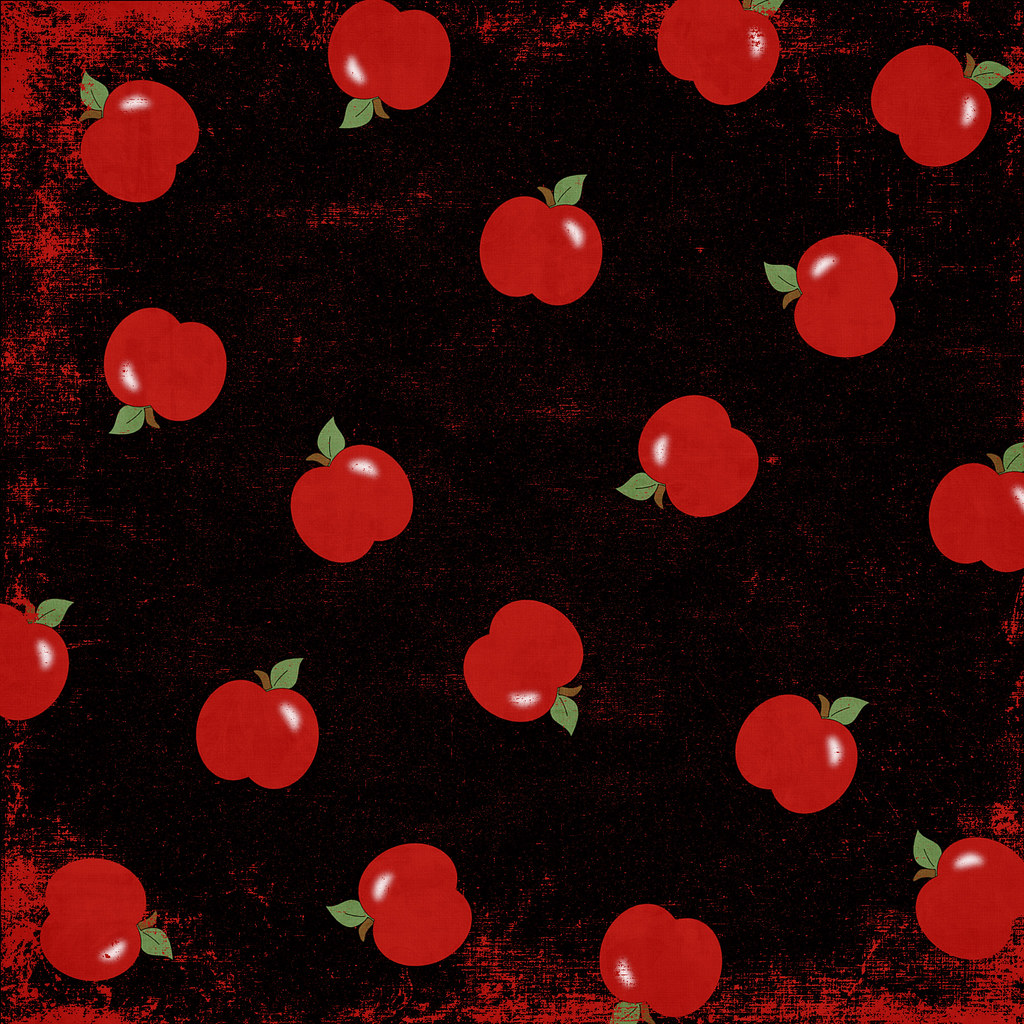The image is a square graphical digital artwork dominated by a predominantly black background with subtle streaks and splashes of red, particularly prominent towards the upper left, lower left, and lower right areas. Scattered across this backdrop is a repeating pattern of identical, glossy red apples, each featuring a brown stalk curving to the left and a green leaf pointing towards the top right diagonal. The apples are orientated in various directions—some facing upwards to the left corner, others tilted to the right, and some even upside down—creating an evenly spaced, sporadic arrangement that resembles a step-and-repeat pattern often used in advertising or media. The highlight or light bounce on each apple, situated in the top right corner if correctly oriented, adds a realistic touch to the otherwise simplistic, cartoon-like depiction, making the whole image appear as though it could serve as a whimsical wallpaper design or a fabric print.